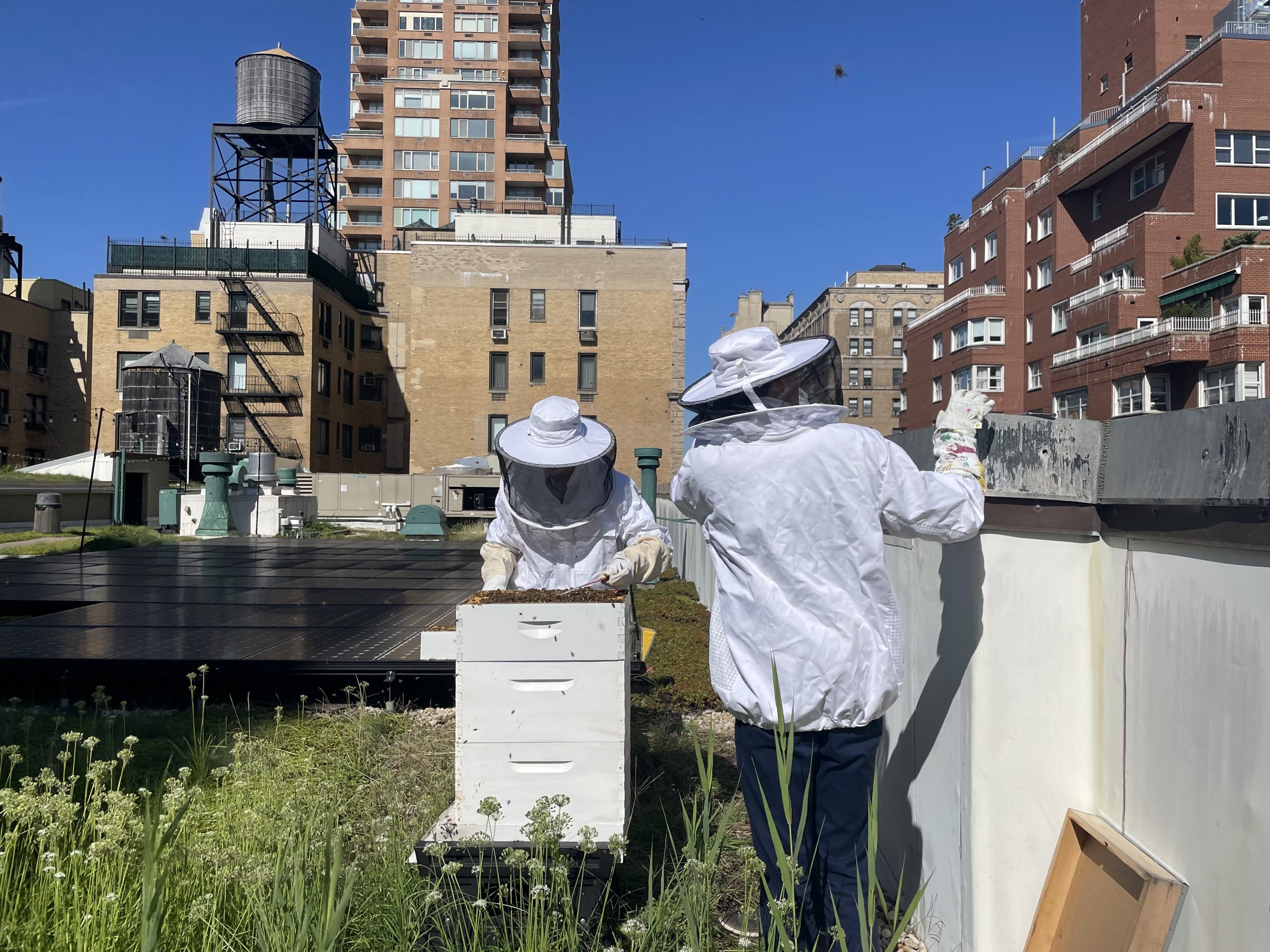The image depicts a pair of beekeepers working on the rooftop of a city building, under a bright, clear sky with no clouds. Both beekeepers are clad in full white protective suits, including gloves and headgear to shield themselves from the bees. One beekeeper, on the left side of the image, is intently tending to a white bee box containing shelves filled with bees. The second beekeeper, positioned on the right, appears to be observing their partner’s work while also standing near solar panels and an empty bee box. Behind the beekeepers, the city's skyline is visible, featuring a mix of red and brown brick buildings, tall apartment structures, and a water tower. The rooftop is adorned with green grass and scattered flowers, providing a natural habitat for the bees. Additionally, typical rooftop fixtures such as AC units are seen, reinforcing the urban setting of this unique beehive location.